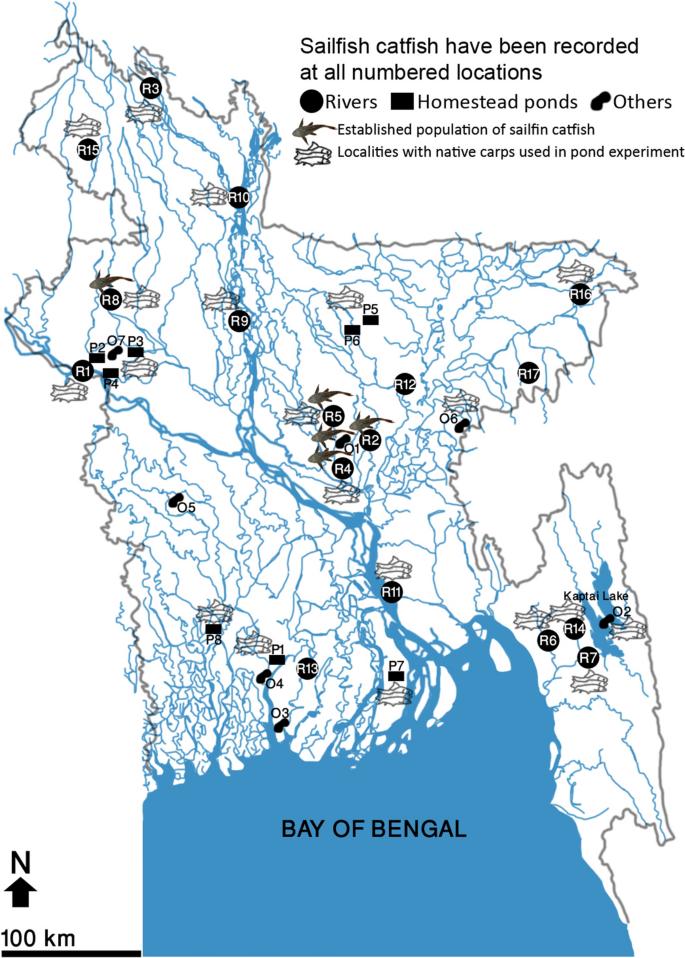This detailed infographic showcases a map of Bangladesh and the Bay of Bengal, illustrating the distribution of sailfish catfish at various locations. The map is predominantly colored in shades of white, blue, black, and gray. At the top right-hand corner, there is text stating, "Sailfish catfish have been recorded at all numbered locations." Accompanying this statement is a key that deciphers the map's symbols: round black circles representing rivers, black squares for homestead ponds, and two small circles denoted as 'others.' 

The map also highlights an established population of sailfish catfish, depicted with fish icons, and indicates localities where native carps are used in pond experiments with boat icons. The blue lines on the map symbolize the rivers winding through Bangladesh, complemented by a myriad of circles and squares pinpointing specific spots where these observations have been made. At the bottom, labeled in dark blue, is the Bay of Bengal, providing a clear geographical reference. Additionally, in the left-hand corner, there is a navigational arrow with an "N" signifying north, and a scale that reads "100 KM," enhancing the map's readability and accuracy.